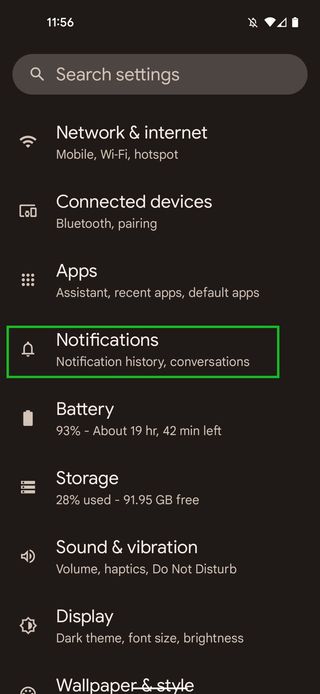The image depicts an overview of settings in an Android app presented in dark theme mode, featuring a black background with white text. At the top, there is a search bar allowing users to search within the settings. Below the search bar, a list of categories is displayed in a vertical arrangement: 

1. **Network & Internet** with subcategories such as Mobile, Wi-Fi, and Hotspot.
2. **Connected Devices**
3. **Apps** with options like Assistant, Recent Apps, and Default Apps.
4. **Notifications** (highlighted with a green outline indicating an edited focus perhaps for instructional purposes).
5. **Battery**, showing a level of 93% with an estimated remaining time of about 19 hours and 42 minutes.
6. **Storage**, illustrating 28% usage with 91.95 GB free.
7. **Sound & Vibration**
8. **Display**, where it's clear that the dark theme is enabled, with additional settings for font size and brightness.
9. **Wallpaper & Style**.

Each category is accompanied by descriptors providing additional context. The highlighted green box around "Notifications" suggests somebody is emphasizing or explaining a setting within that section.